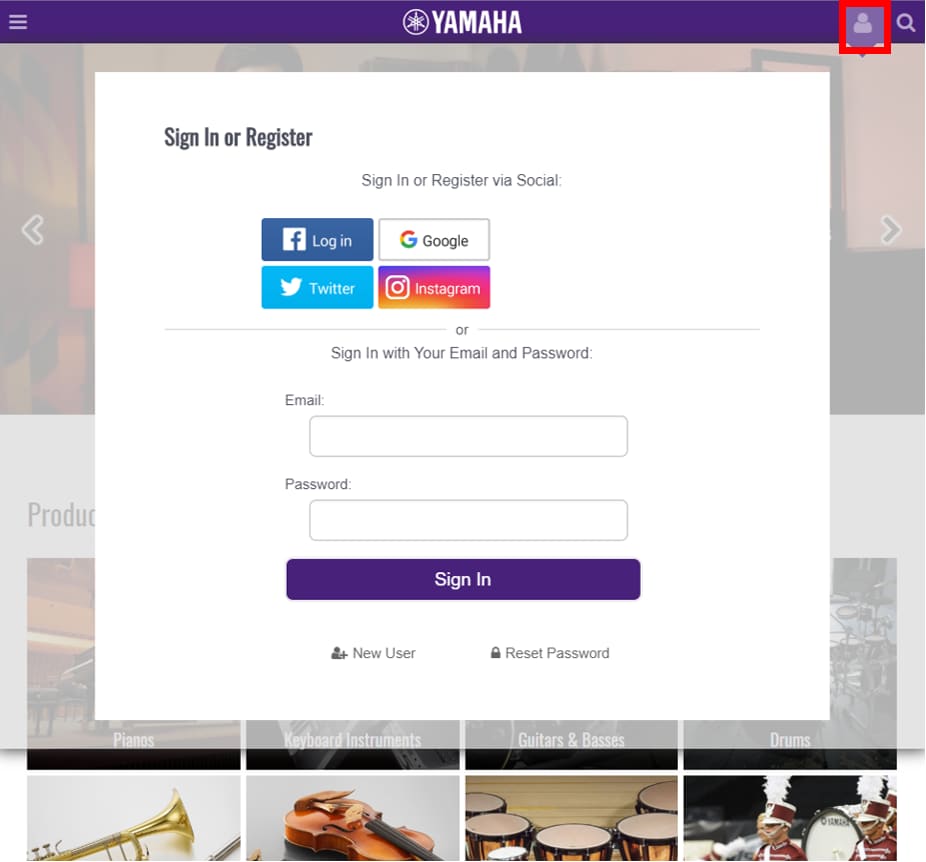This image captures a computer screen displaying a Yamaha webpage. At the top of the screen, there's a prominent purplish rectangle featuring the Yamaha logo and a circular emblem next to it. In the upper right corner, a silhouette of a person is highlighted with a red overlay. Below this, there is a search bar iconified by a magnifying glass.

The central portion of the screen displays a section for user authentication. It prominently features options to "Sign In or Register" marked with the heading "Via Social," offering buttons for logging in with Facebook, Twitter, Google, and Instagram. Below a faint gray divider, the screen provides an alternative login method with the text "Or," followed by fields for email and password entry. Finally, at the bottom, there is a "Sign In" button in a navyish purple color.